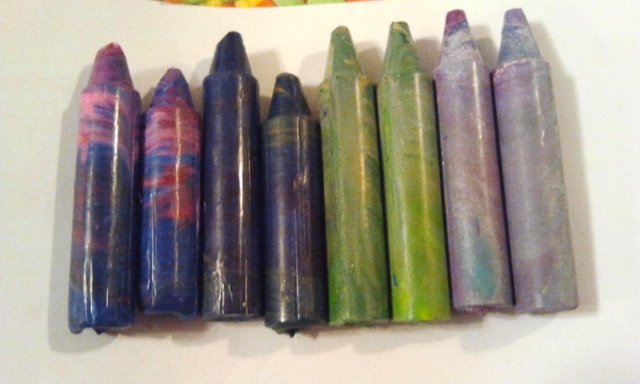This photograph, likely taken in an art studio or art class, showcases eight crayon-shaped, wax-like objects arranged in a row on a white piece of paper, which forms the background for the majority of the image. The crayons display an array of vibrant and non-traditional colors, giving them a tie-dye appearance. From left to right, the first two feature a blend of blue and red; the next two are primarily dark blues and purples with touches of yellow and green; the following pair ranges in shades of green and yellow; and the final two exhibit light purples and violets with hints of aqua, white, and possibly pink. The background slightly visible in the upper portion of the photo includes splashes of yellow, orange, and green. Soft shadows cast by the crayons extend to the bottom left, adding depth to the composition.